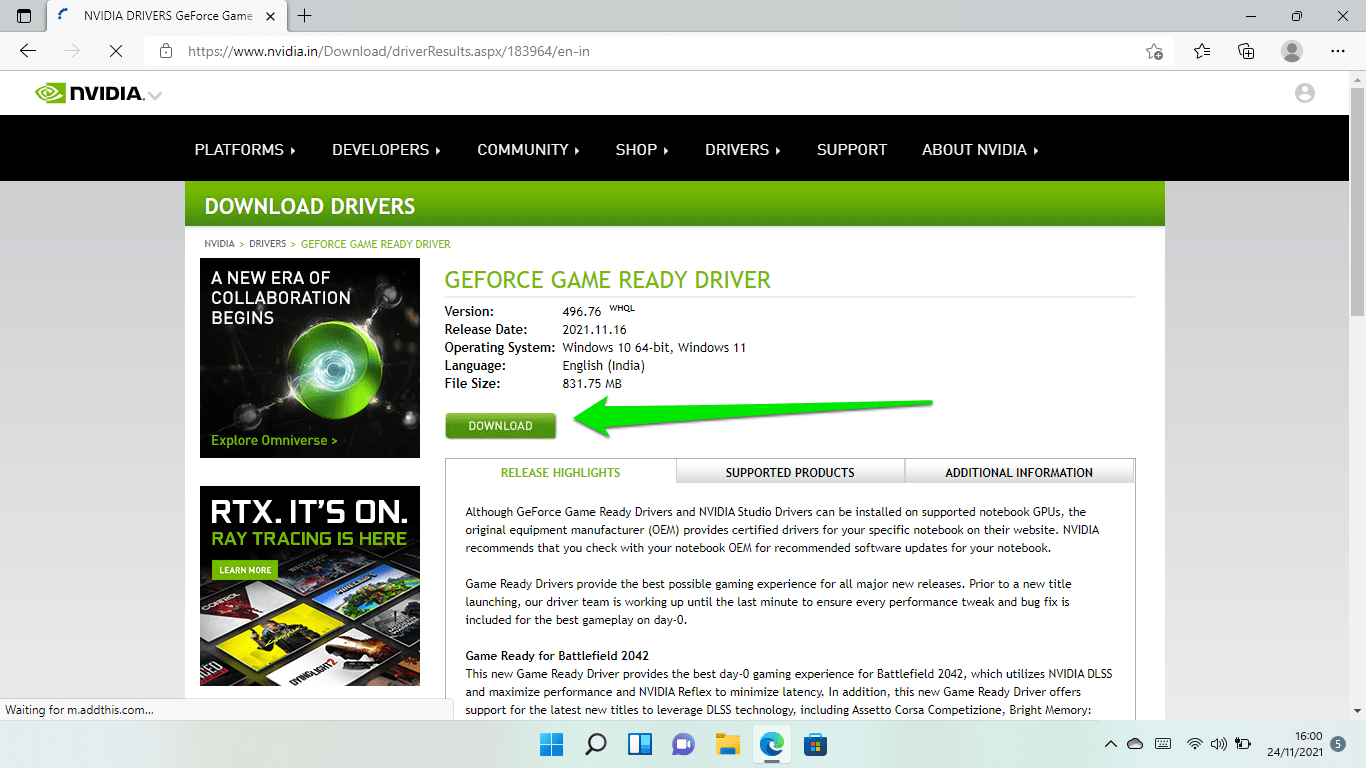This detailed caption describes a screenshot of a webpage from NVIDIA's official website. The top navigation bar contains links labeled "Platforms," "Developers," "Community," "Shop," "Drivers," "Support," and "About NVIDIA." Below this, there is a prominent section for downloading drivers, specifically highlighting the "GeForce Game Ready Driver." The accompanying text introduces a new era of collaboration with a focus on the "Omniverse version 496.76." The detailed information provided includes the tiny-print release date of 2021-11-16, compatibility with Windows 10 (64-bit) and Windows 11 operating systems, the language setting "English (India)," and a file size of 831.75 MB. There is a green arrow icon indicating the download option, followed by release highlights and further information on the installation process of GeForce Game Ready drivers and NVIDIA Studio drivers.